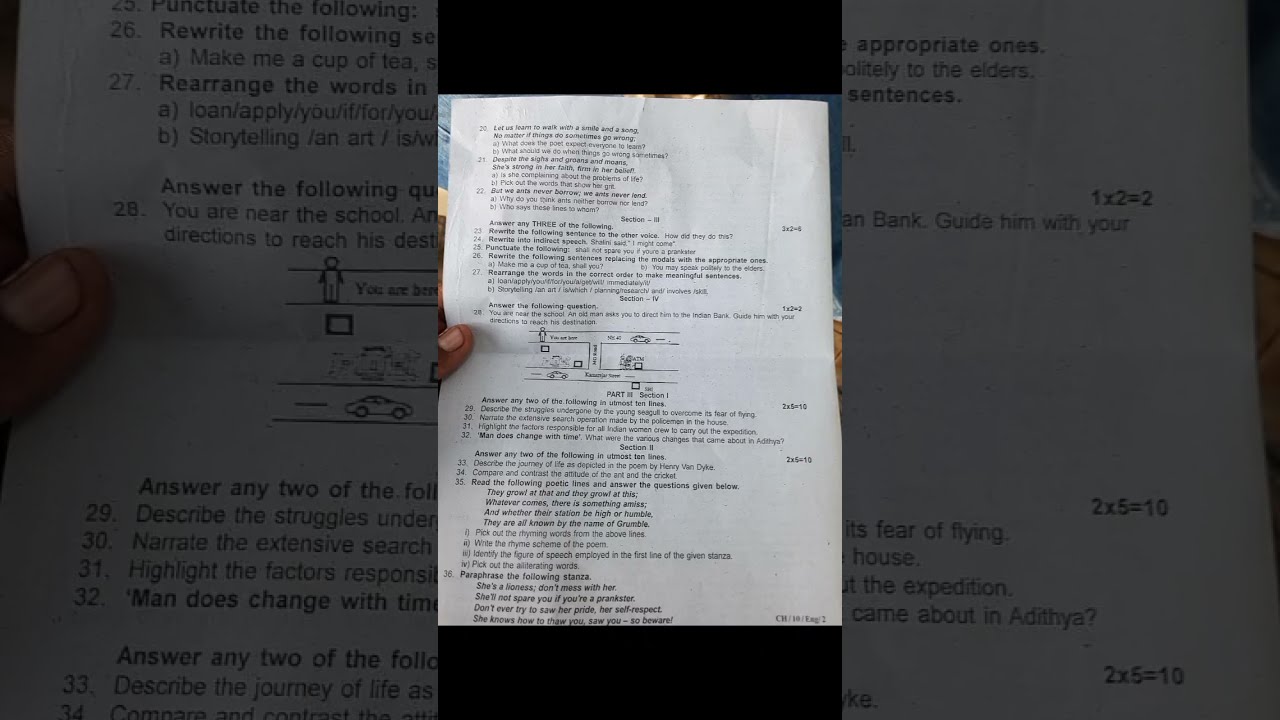The image depicts a piece of white paper densely packed with black text, being held in a person's left hand, likely a quiz or test document. The numbers on the paper range from 20 to 36, indicating a series of sequential questions. The majority of the questions are followed by multiple-choice options. Notably, question 28 includes a small diagram resembling a road, which comes with associated questions. You can see the person's thumb near this question, indicating where the hand grips the paper. The text on the paper covers various scenarios, featuring literary analysis, such as interpreting a poem, and perhaps some questions related to understanding language. Additionally, there are numerical equations on the right-hand side, suggesting a mix of subjects, possibly indicative of a general knowledge or comprehensive test. The paper contains detailed, open-ended questions like "What does the poet expect everyone to learn?" and "Why do you think ants never borrow or lend?" near the top of the list, highlighting its nature as an evaluative educational tool.